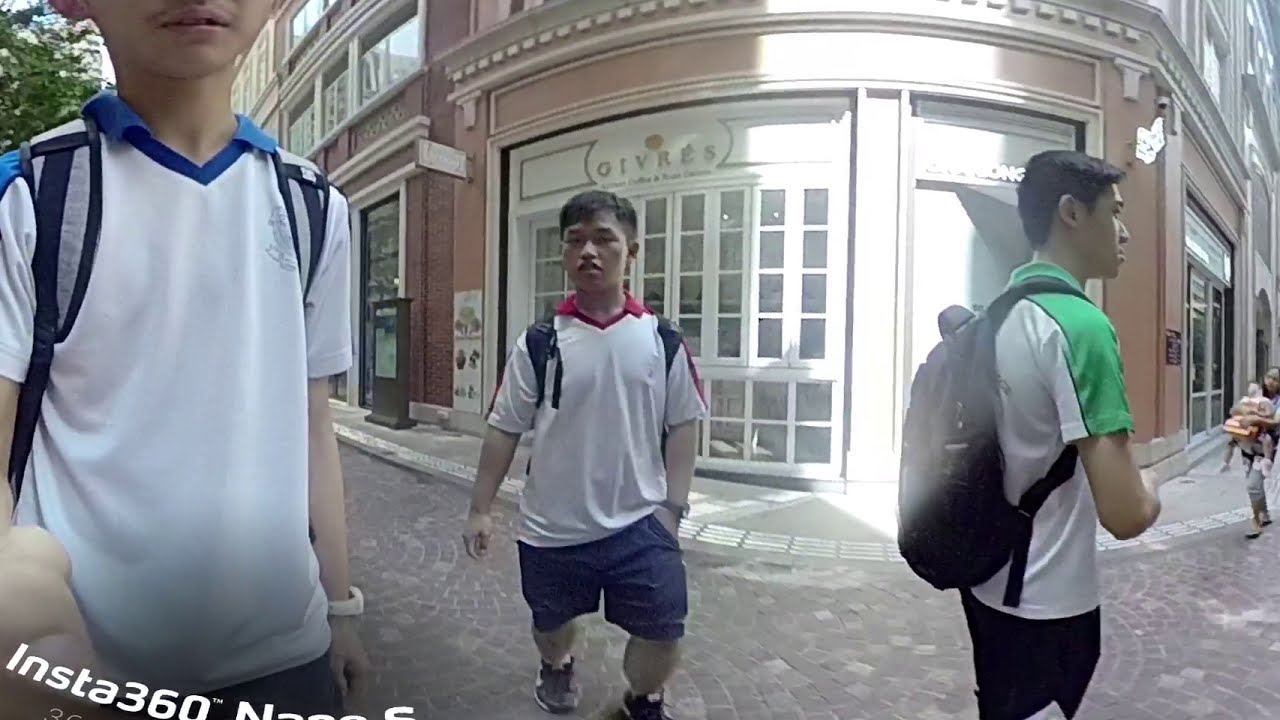In the photograph, a vibrant city street scene during daylight is captured in a wide-angle, panoramic shot. Central to the image are three young Asian men, likely in their teens or early twenties, standing on a cobblestone-paved street. Each man is wearing a white jersey-style shirt with distinct colored trims — red, blue, and green respectively — paired with shorts and backpacks. The man in the center sports a white shirt with red trim and black shorts, holding a backpack with black straps. To the left, another man is seen in a white shirt with blue trim and black and gray backpack straps, noticeable as he is also wearing a watch. On the right, the third man is dressed in a white shirt with green trim and carries a gray backpack, also wearing black shorts. In the background, the elegant scenery continues with a storefront displaying the sign "GIVRES" in gold letters atop a brick facade with white-framed window panels. The surroundings suggest an upscale section of the city, emphasizing the ornate and neatly maintained environment. Additionally, in the lower left corner of the photo is the text "INSTA360" along with the letter "N," hinting at the panoramic nature of the image. Lastly, the right edge of the photograph captures a glimpse of another person wearing distressed jeans, walking towards the three men.